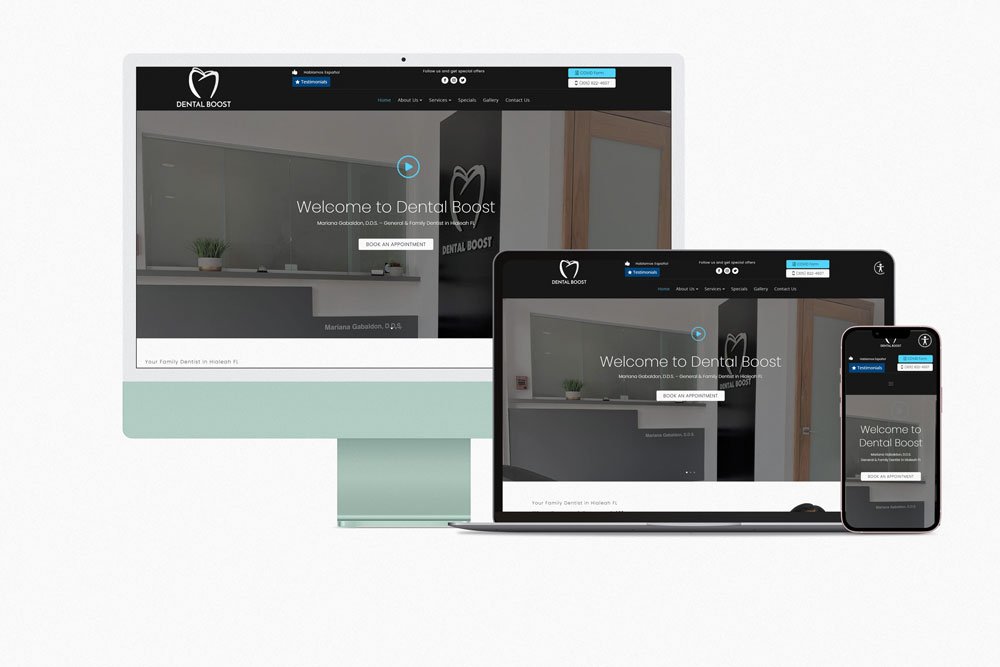In this image, three electronic devices are prominently displayed in close proximity to each other. Positioned on the left is a computer monitor, characterized by a mint green color. In the center is a laptop, and to its right rests an iPhone. All three screens showcase the same online interface, which features the text "Welcome to Dental Boost."

The design details are consistent across the devices with a significant amount of visual coordination. In the top left corner of each screen, the logo for Dental Boost is visible, stylized to resemble a heart. At the center of the display on all devices, there is a prominent blue, circular play icon, located directly above the welcoming text. This cohesive presentation underlines the uniform accessibility and consistent branding of the Dental Boost website across various digital platforms.